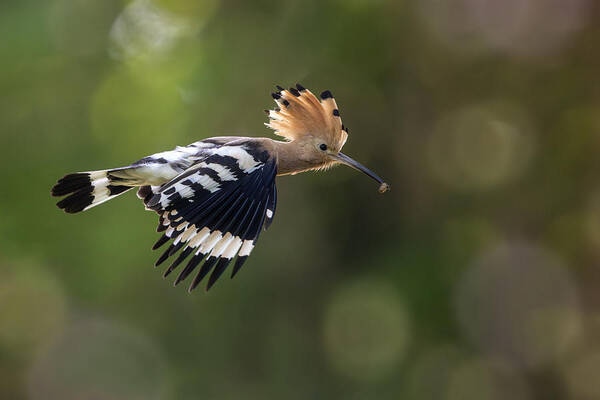The photograph captures a vibrant image of a Eurasian hoopoe in flight, set outdoors during the day under natural light. The composition is an intriguing combination of horizontal and vertical elements, featuring a blurred, primarily green background with various patches of lighter hues, possibly illuminated by sunlight filtering through foliage. The bird, flying towards the right side of the frame, is distinguished by a notably long, thin black beak and a unique crown of tan-brown feathers tipped with black, giving it a punk rock appearance. The hoopoe's body exhibits a striking contrast of black and white stripes, particularly on its wings, where a prominent white stripe does not quite reach the tip. Its tail mirrors this pattern with black and white stripes. The fast shutter speed of the camera has perfectly frozen the motion of the bird, from the defined feathers to the potential worm or object dangling from its beak. The overall clarity of the bird against the softly blurred backdrop emphasizes the dynamic energy and vivid detail of the scene.